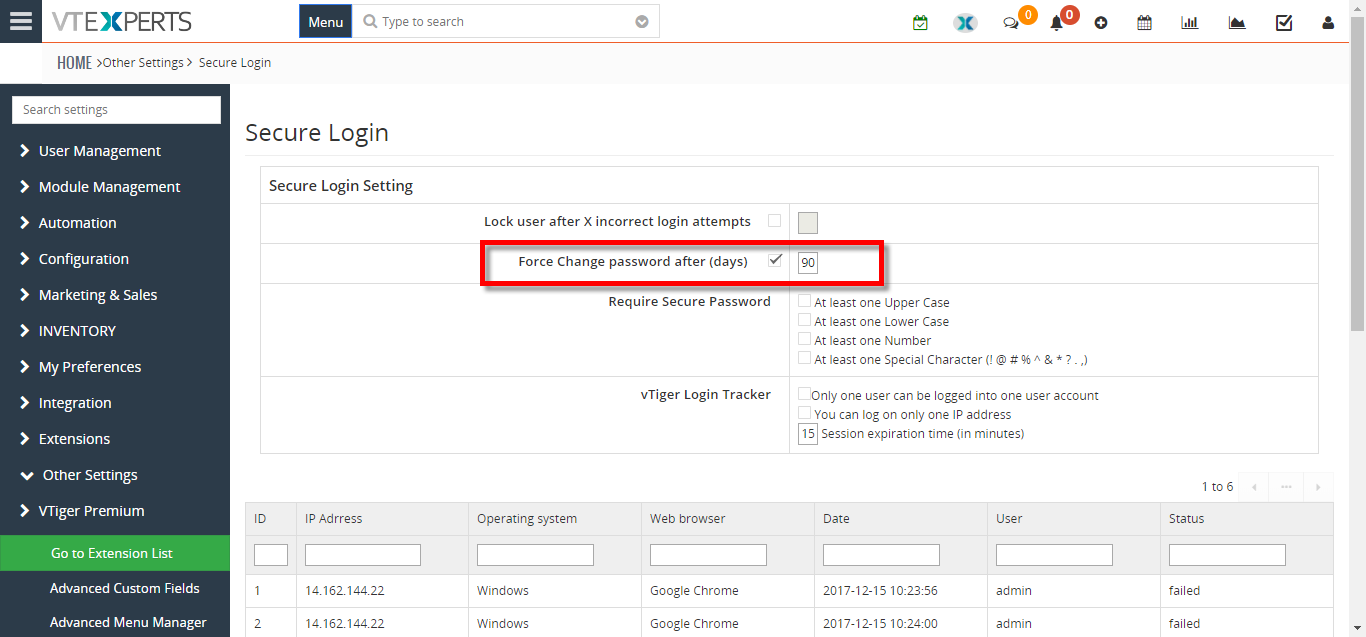The screenshot captures a website interface, showcasing various elements clearly and in detail. 

In the upper left-hand corner, there is a button featuring three horizontal lines stacked on top of each other, set against a dark black-grey background. To the right of this button, the brand name "VTExperts" is displayed, with the "X" in blue. Further to the right, there is a button labeled "Menu" in white text on a black background, possibly with a blue border or an extended border, although this is unclear.

Next to the "Menu" button is a magnifying glass icon, representing the search function, accompanied by a "type to search" text box. Adjacent to the search box is a down arrow within a gray circle. To the far right, there is a series of icons.

Below this header section, there is a breadcrumb navigation trail, indicating the user's path through the site: "Home > Other Settings > Secure Login."

The screenshot also displays a dual-column layout. The left column serves as a sub-menu, listing various options in the following order: "Search Settings," "User Management," "Module Management," "Automation," "Configuration," "Marketing and Sales," "My Preferences," "Integration," "Extensions," "Other Settings," "VTiger Premium," and a sub-menu highlighted in green titled "Go to External List." Below this are items such as "Advanced Custom Fields" and "Advanced Menu Manager."

The right column contains a section for "Secure Login," followed by "Secure Login Settings," with several labeled input fields. Further down, there are multiple columns and rows displaying a header and at least two rows of information.

Overall, the screenshot provides a comprehensive view of the website's navigation and configuration options, structured neatly into distinct sections and sub-menus.